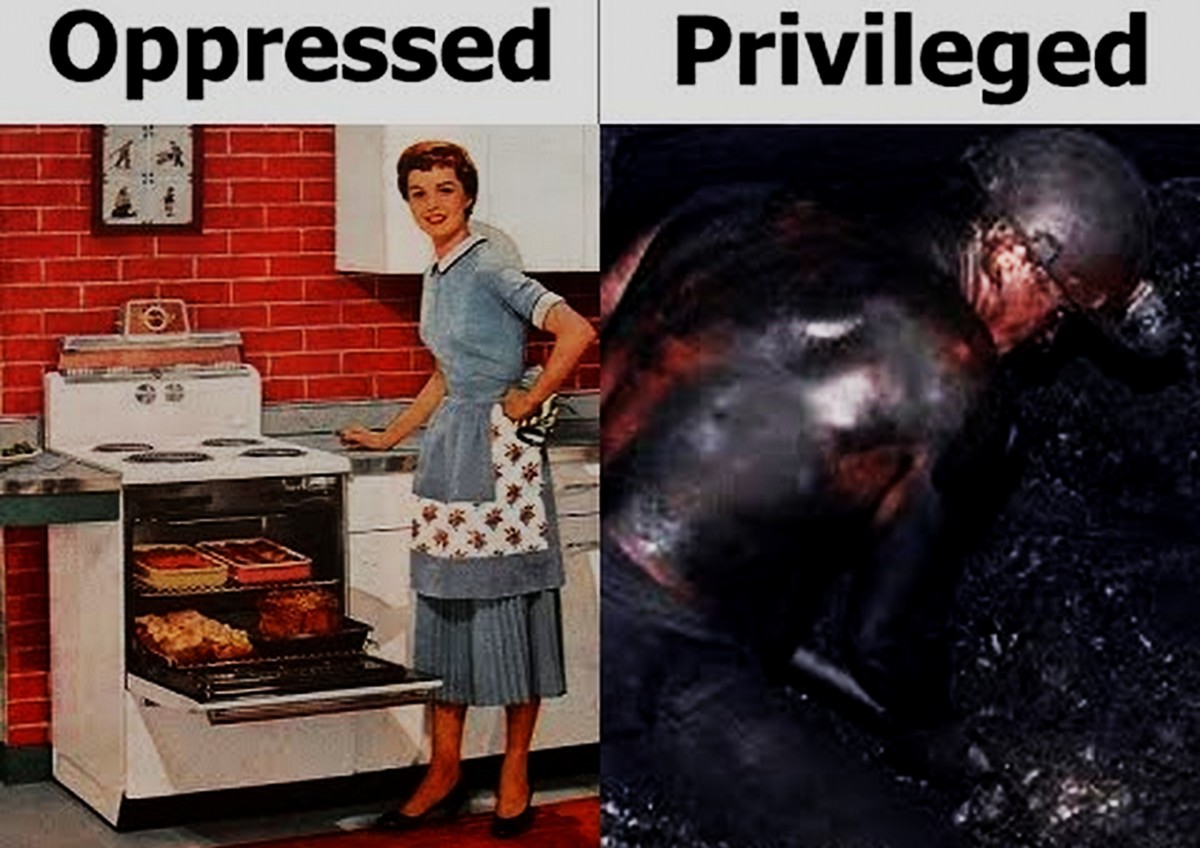This two-part meme uses sarcasm to comment on societal roles. On the left side, labeled "oppressed," there is an illustration of a 1950s-style woman in a kitchen. She is wearing a white flowered apron over a grey outfit with a white collar and skirt. She stands by an open electric oven, cooking multiple dishes including a large roast and casseroles, and looks directly at the viewer. On the right side, labeled "privileged," is an image of a shirtless man, covered in black oil or soot, wearing a helmet with a flashlight. He appears to be engaged in strenuous manual labor, possibly as a coal miner. The juxtaposition of the clean, domestic scene with the dirty, physically demanding work serves to highlight the ironic use of the terms "oppressed" and "privileged."